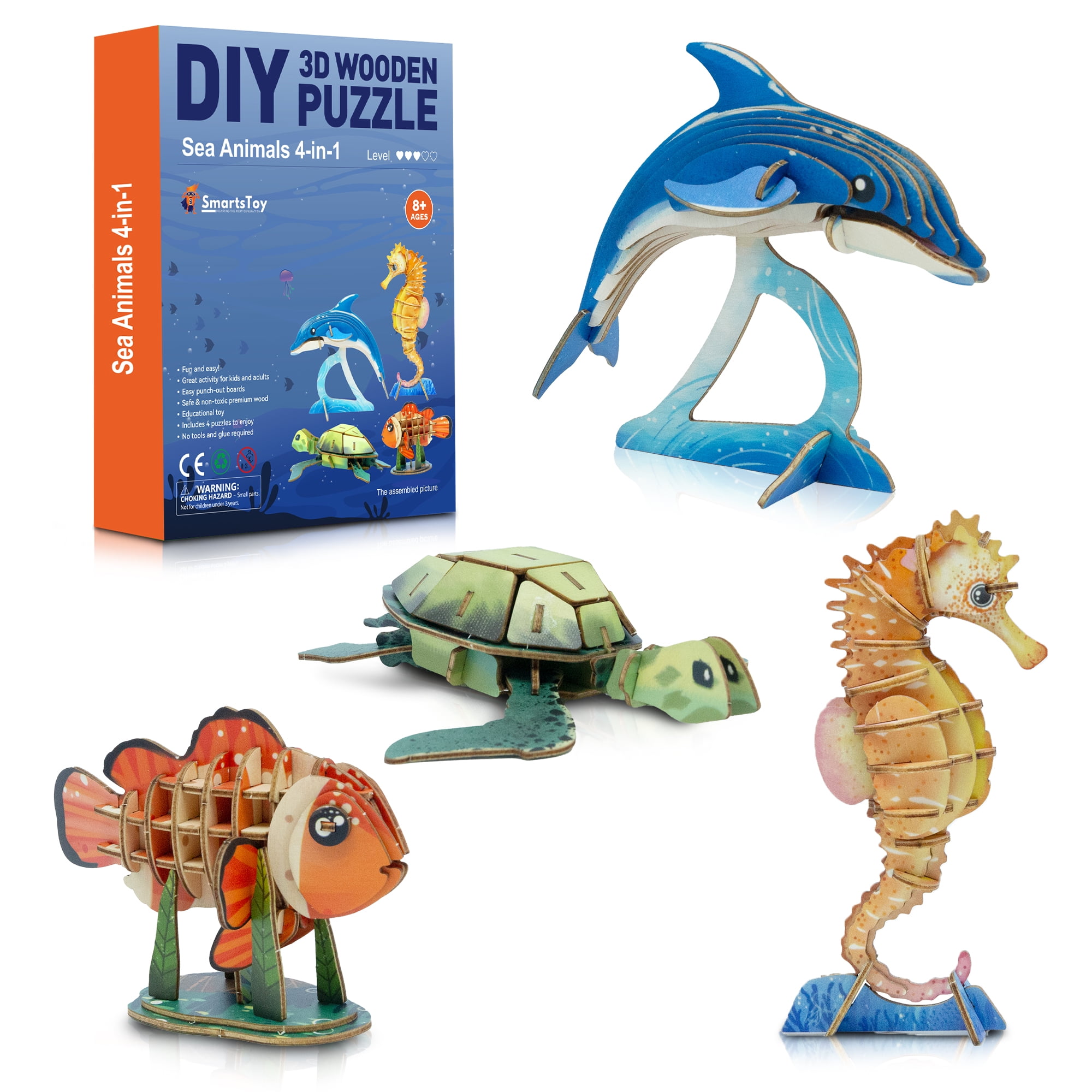The image showcases a vibrant DIY 3D wooden puzzle set titled "Sea Animals 4-in-1." The top left corner of the image shows the product box, which has a blue and orange design featuring an ocean background. The box text reads "DIY 3D Wooden Puzzle, Sea Animals 4-in-1, Level" with three hearts filled and two empty, along with "Smarts Toy" and "Ages 8+".

The set includes four exquisitely detailed sea animal figurines: a blue and white dolphin, a light green turtle, an orange and yellow seahorse, and an orange and white clownfish. Each animal is constructed from layered wood pieces, giving them a 3D puzzle-like appearance.

1. **The Dolphin:** Mounted on a light blue, wave-shaped stand, the dolphin features a blue top and a white underbelly, with black eyes, giving it a lifelike appearance of leaping out of the water.
2. **The Turtle:** This green turtle with black eyes is depicted lying flat on the ground, without a stand. Its outstretched flippers give it a serene, swimming posture.
3. **The Seahorse:** Standing upright on a blue pedestal, the seahorse is predominantly orange with yellow accents and dark blue eyes. It features ridge lines across its body and a curled tail which elegantly elevates it.
4. **The Clownfish:** Featuring a vibrant combination of orange with white stripes, the clownfish rests on a green stand with four prongs, resembling ocean coral or sea grass.

The figurines are shown in simultaneous assembly and completed states, highlighting their intricate detailing and the layered wood texture. The overall impression is colorful and lively, perfectly capturing the essence of marine life.